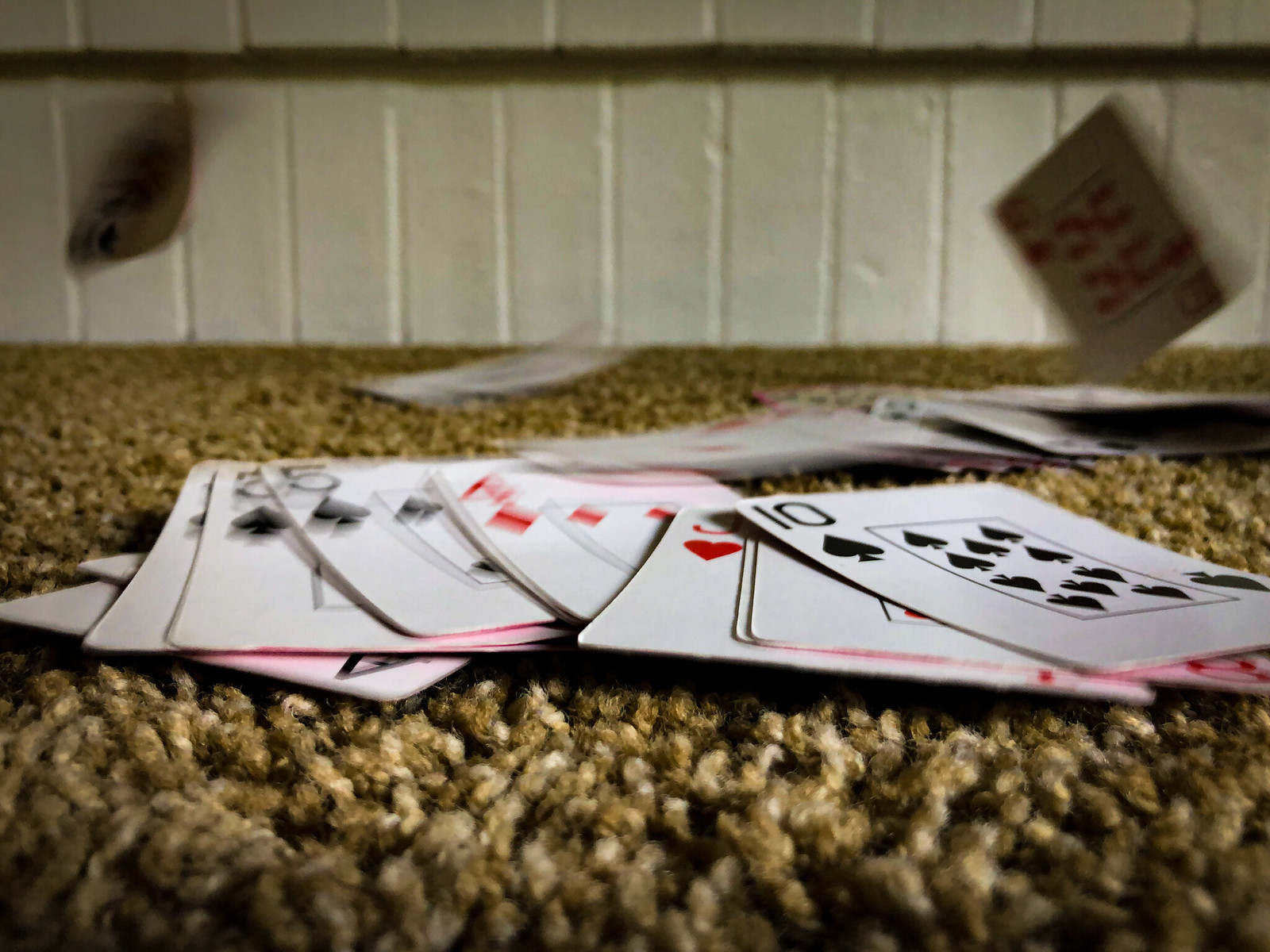The image captures a dynamic scene of playing cards scattered across a brown and white patterned carpet. In the foreground, a distinct arrangement of cards including an Ace, 3, 4, 5, and 10 is clearly visible on the floor. The background adds a sense of motion with multiple cards appearing to fly, captured mid-air and slightly blurred to emphasize their swift movement. The left side features a noticeably motion-blurred card, enhancing the dynamic effect. The scene is set against a backdrop of a white brick wall and is illuminated with moody lighting, creating a dramatic and somewhat mysterious atmosphere. The viewpoint of the image is from a low angle close to the floor, adding depth and a unique perspective to the composition.